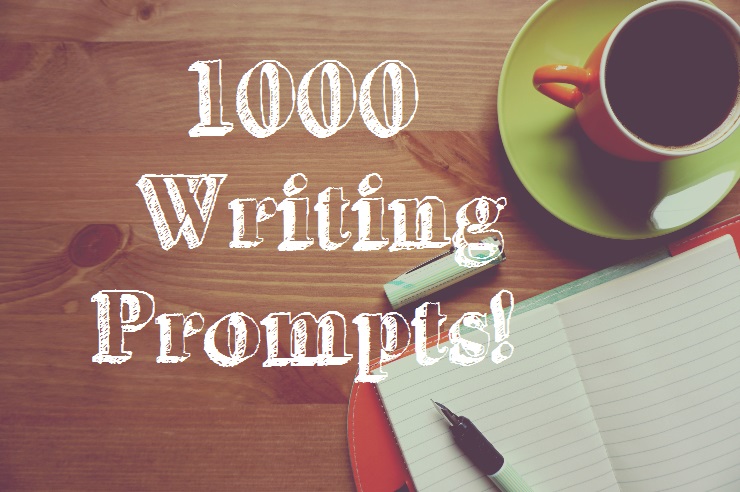The image depicts a light wood table that serves as the backdrop for several objects designed to inspire writing. In the upper right corner, a vibrant green saucer holds an orange coffee cup, adding a splash of color to the scene. Below this, toward the lower right, an open notebook with blank pages lies ready for use. Placed atop the left page of the notebook is a pen, with its cap resting nearby. To the left side of the image, three lines of white text are graphically designed to read "1,000 writing prompts," suggesting the purpose of the items on the table. The combination of these elements creates an inviting atmosphere for creativity and reflection.